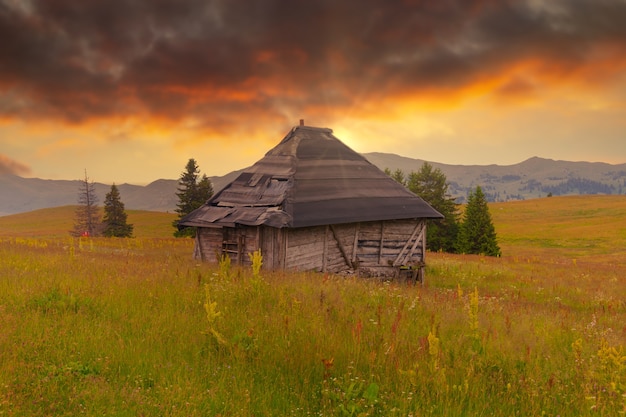The image depicts a painting of a small, weathered wooden shack situated in a vast field of tall grasses that are a mix of yellow, green, and patches of red. The shack appears run down, with tan and gray colored wood that looks warped and potentially abandoned, as the windows seem boarded up and the roof has noticeable gaps, particularly on the side facing left. The landscape is dotted with a few evergreen, cone-shaped trees, and in the background, a mountain range spans the horizon. Above the mountains, the sky is in a state of either sunset or sunrise, transitioning from dark, thick clouds at the top to hues of orange and yellow closer to the mountains. The overall scene is illuminated by a soft, golden light from the sun in the distance, enhancing the sense of tranquility and solitude in this rustic setting.